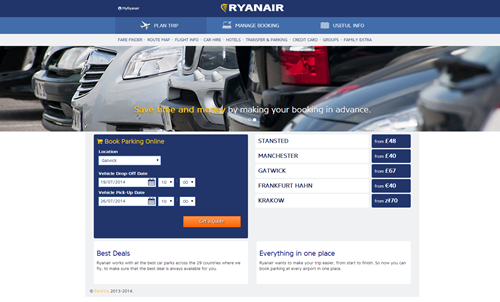The image depicts a small, rectangular webpage that is approximately 50% wider than it is tall, making details somewhat hard to discern. At the top of the webpage is a royal blue bar that spans the entire width and takes up about 10% of the image's height. A centrally positioned logo is present within this blue bar. The logo consists of a capital 'D' shape turned backward, rendered in a yellow-gold font. Next to the logo, aligned to the right, are the bold, all-capital letters "RYANAIR" in white, indicating the airline's branding.

Below this, there is a lighter blue bar of equal height, containing three navigational options. From left to right, the first option is marked by a slightly darker blue, indicating it is the currently selected option. This option features an airplane icon and the text "PLANNED TRIP." The second option displays a bus icon and the text "MANAGE BOOKING," while the third option features a suitcase icon and the barely readable text "USEFUL INFO."

Underneath the navigation bar, there is a black menu bar with approximately eight to ten centered menu options, although the text is not legible. Further down, occupying about a third of the screen's height, is a banner showcasing the front bumpers of several parked cars. At the bottom of the image is a selection tool intended for customizing trip details, although the specific elements of this tool are not readable.